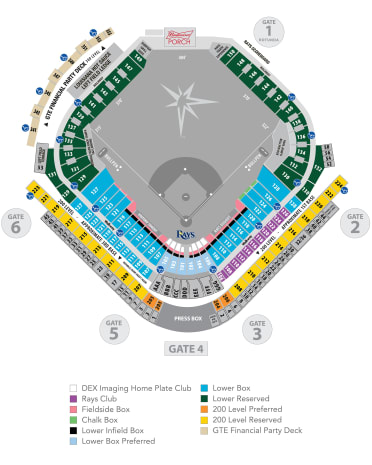The image depicts a detailed seating chart of a baseball stadium. The stadium, identifiable by its distinctive field layout, showcases an expansive seating arrangement colored in a variety of hues. Specific sections include the "DEX Imaging Home Plate Club," "Raise Club," "Field Side Box," "Chalk Box," "Lower Infield Box," "Lower Box Preferred," "Lower Box," "Lower Reserved," "200 Level Preferred," "200 Level Reserved," and the "GTE Financial Party Deck." Each seating area is color-coded in shades of green, white, purple, pink, black, blue, darker blue, darker green, orange, yellow, and tan. The chart also highlights entry gates numbered one through six, strategically positioned around the stadium.

The central field area is uniquely represented in gray, contrasting with the white background encompassing the entire diagram. The legend uses both black and white fonts to denote various sections and provide clarity. Additionally, there are blue circular icons with a "Y" symbol, whose specific purpose is unclear from the description. This seating chart serves as a comprehensive guide for fans, aiding them in ticket purchasing and navigation around the stadium.